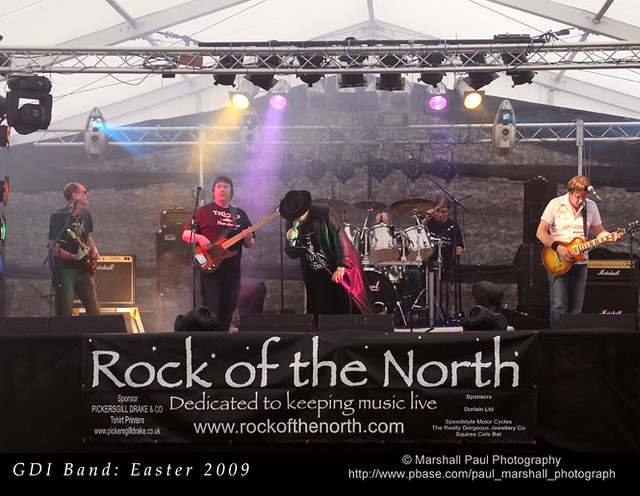The image is a detailed poster of an outdoor concert featuring a live band named "GDI Band" during their performance on Easter 2009. The stage is vibrant with multicolored lights—purple, yellow, and blue hues—illuminating the performers and adding to the energetic ambiance. The band consists of five members: a guitar player on the left, a bass player, a singer in the center, a drummer positioned at the back, and another guitar player on the right. All members face forward, engaging with the audience. In the background, there is text that prominently reads "Rock of the North, dedicated to keeping music live" along with the website "www.rockofthenorth.com." Additional details include the text "Marshall Paul Photography" written in white in the lower right corner, signifying the photographer of the image. The stage itself features hues of black and gray, contrasting with the colorful lights streaming across the band members. Some text elements are quite small and challenging to read, adding a layer of intricacy to the poster's design.